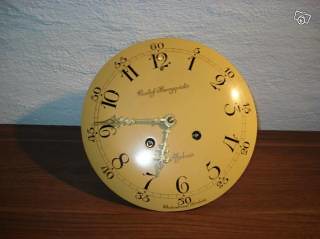This image features a close-up of a minimalist clock face devoid of any rim or ring, showcasing only the solid metal surface. The clock has a yellow base and is equipped with gold hour and minute hands, currently indicating the time as 14 minutes to 7. The dial is marked with numbers ranging from 1 to 12, with intervals of five minutes annotated around the circumference (e.g., 5, 10, 15, 20, etc.). Cursive text is visible beneath the 12 o'clock position and above the 6 o'clock position, though the writing is indistinct. The clock is situated on a wooden table, set against a white, rough-textured wall.